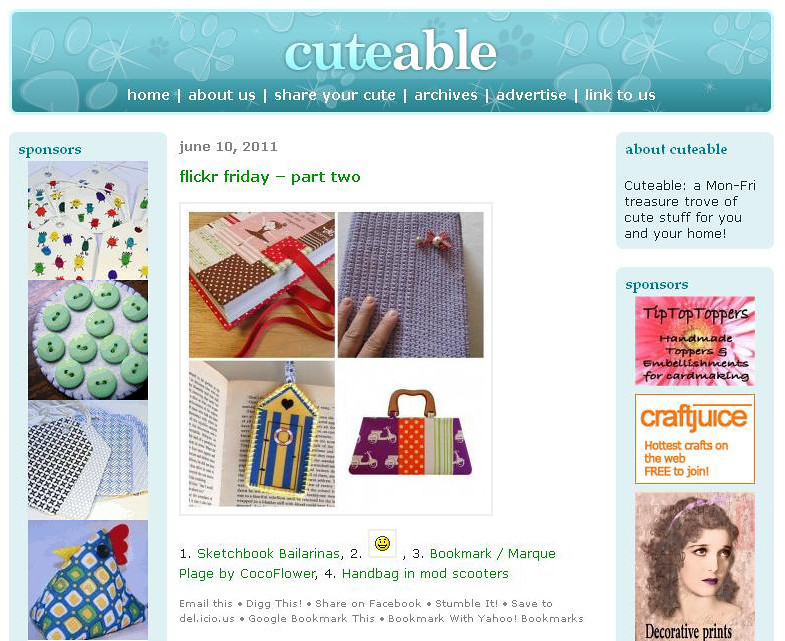The image depicts a colorful homepage of the website "Cutable," featuring a light blue banner at the top adorned with paw print designs. In the center of the banner is the title "Cutable." Beneath the banner is a navigation bar with the links: "Home," "About Us," "Share Your Cute," "Archives," "Advertise," and "Link to Us." 

On the left-hand side of the page, there is a vertical pane labeled "Sponsors," which displays photographs of various decorative and clothing items. The center of the page prominently features the date "June 10th, 2011," and the title "Flickr Friday Part 2," below which are four images of colorful fabric and decorative products. Additionally, underneath this section, different items are listed: "Sketchbook Ballerinas," "Bookmark Mark/Marque," "Plague by Cocoa Flower," and "Handbag in Mod Scooters."

On the right-hand side, a vertical pane labeled "About Cutable" describes the site as "a Monday through Friday treasure trove of cute stuff for you and your home." Below this, the sponsors are listed again: "Tick Tock Toppers," "Craft Juice," and "Decorative Prints." At the bottom of the main section, social media and sharing options are available, including "Email This," "Dig This," "Share on Facebook," "Stumble It," "Save to DEL.ICIO.US," "Google Bookmark This," and "Bookmark with Yahoo."

The page is organized and vibrant, creating a clear and engaging visual presentation for users.